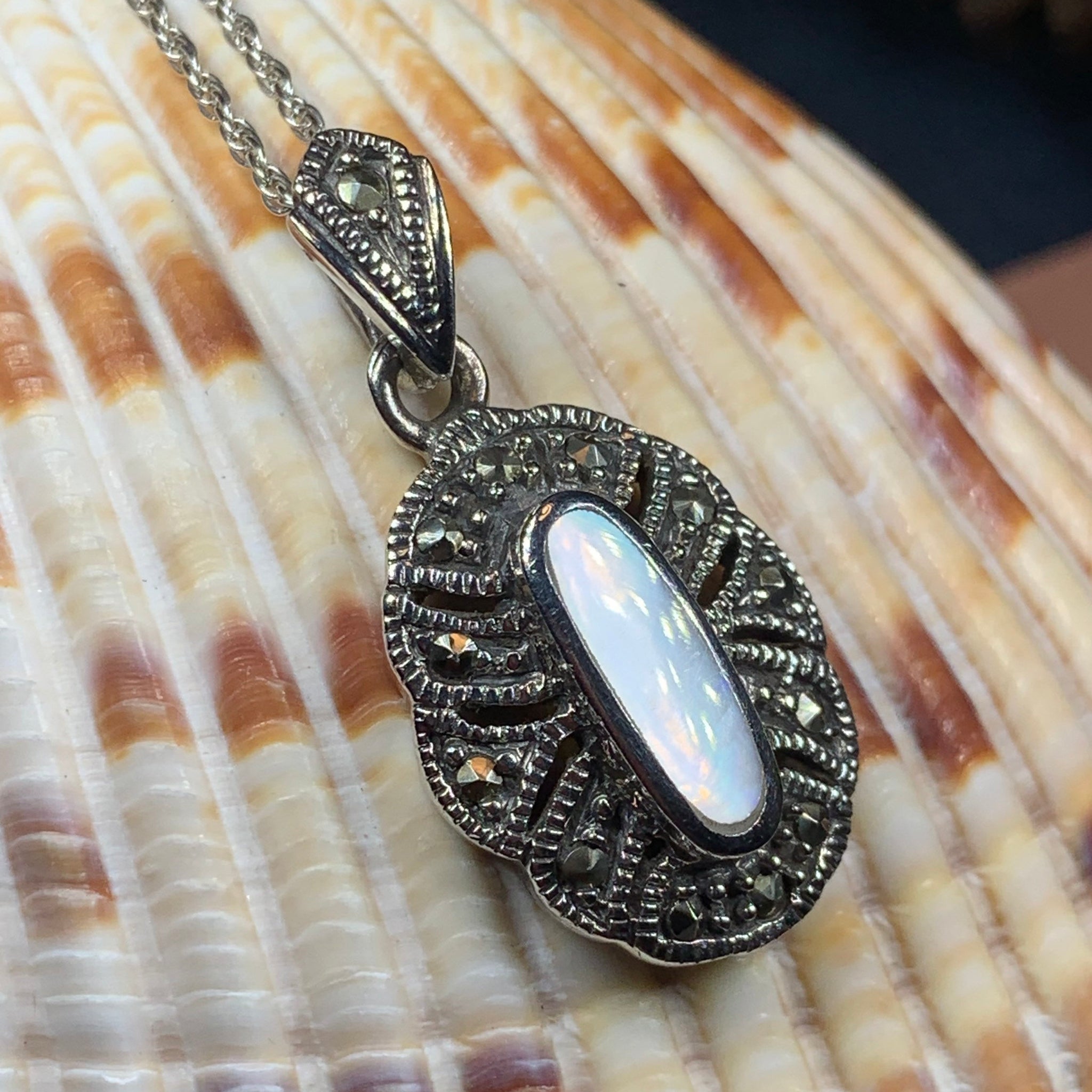This close-up photograph, square in shape at approximately six inches by six inches, features an exquisite necklace elegantly draped over a large seashell. The seashell, exhibiting a captivating pattern of cream and brown stripes with white recessed edges, provides a contrasting backdrop that accentuates the intricate details of the jewelry. 

The necklace, predominantly silver in color, is elegantly poised from a delicate chain that begins at the top of the image and leads to a prominent pendant. The pendant, an oval-shaped charm, showcases a semi-transparent, milky white, and blue stone, polished to a shiny finish. Encircling this central gem is an elaborate metalwork of darker silver, giving the piece an antique appearance.

The composition is meticulously crafted, with the shell’s bands of cream and brown stripes drawing the eye towards the pendant, while the silver chain gracefully drapes, highlighting the necklace's refined elegance. The background of the photo is slightly out of focus, blending into blurry shades of black and brown, ensuring that the ornate necklace and its seashell pedestal remain the captivating focal points, possibly displayed either as part of a personal collection or in a coastal-themed jewelry shop.